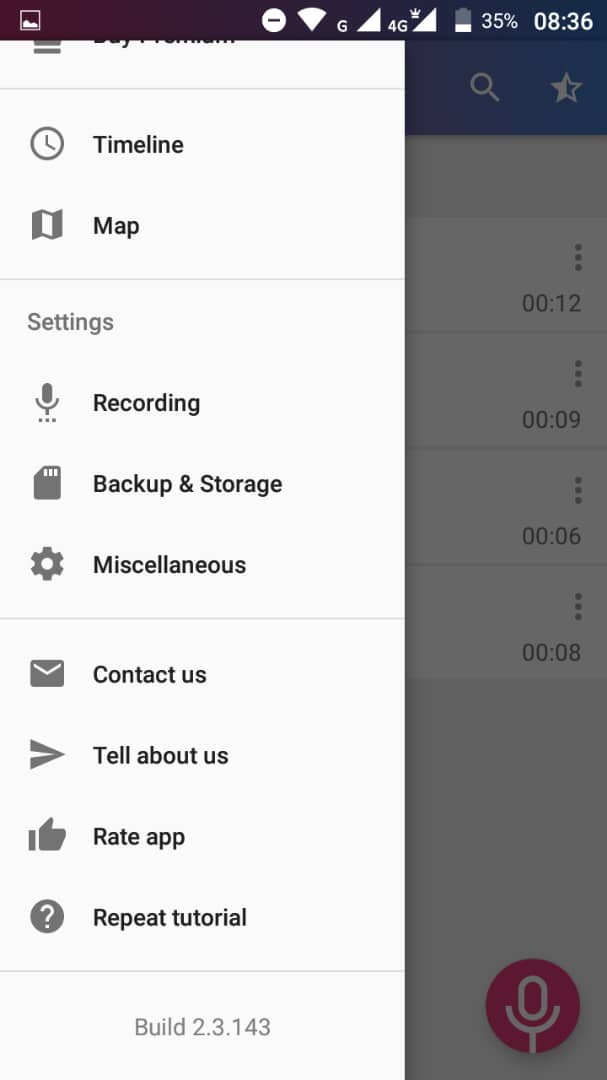The top bar of the interface features a gradient transitioning from a dark red color on the left to a dark blue color on the right. Indicators on the top bar show the battery life at 35%, a 4G connection, and the current time at 8:36. 

On the left side of the screen, there is a long vertical white rectangle containing various menu options, each accompanied by an icon:
- The first option is labeled "Timeline" with a clock icon beside it.
- The second option is "Map."
- The third option is "Settings."
- Beneath "Settings" there is "Recording," with a microphone icon to the left.
- Following that is "Backup and Storage," featuring a disk icon.
- Next is "Miscellaneous," indicated with a turn wheel icon.
- Further down is "Contact Us," depicted with an envelope icon.
- The next entry is "Tell About Us," indicated by an arrow pointing to the right.
- Following that is "Rate App," with a thumbs up icon.
- Finally, there is "Repeat Tutorial," symbolized by a gray circle with a question mark inside.

Below this list, in light gray text, the build version "2.3.143" is displayed. On the right side of the screen, towards the bottom, a red circle icon with a speaker or microphone symbol is visible, likely related to volume controls or voice commands.